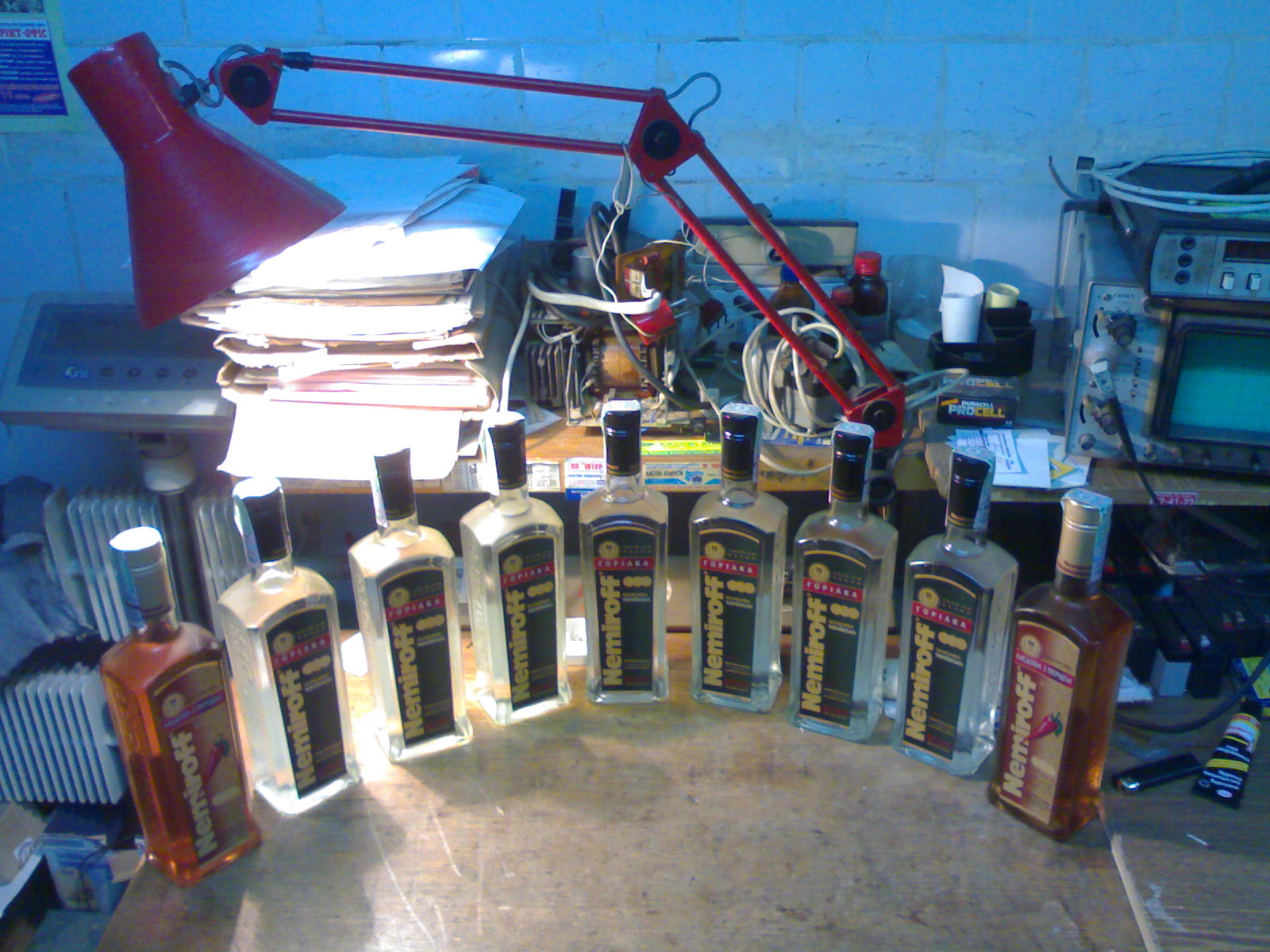The photograph showcases a collection of nine Nemiroff vodka bottles neatly arranged in a curved, outward semi-circle fashion. Seven of these bottles contain clear liquid, while the two bottles at each end hold a brownish-red liquid, likely indicating a chili flavor due to the pepper depicted on their labels. The labels on all the bottles feature Nemiroff's branding in gold with black labels and a red slash going through it. The scene is illuminated by a large, red table lamp that casts light on the left half of the bottles. Situated on what appears to be a wooden desk, the setup also includes various items such as a stack of papers, electrical cords, an old type monitor, metallic radiators, a scale, a lighter, and a bottle of glue, adding a sense of clutter and functional use to the background environment.